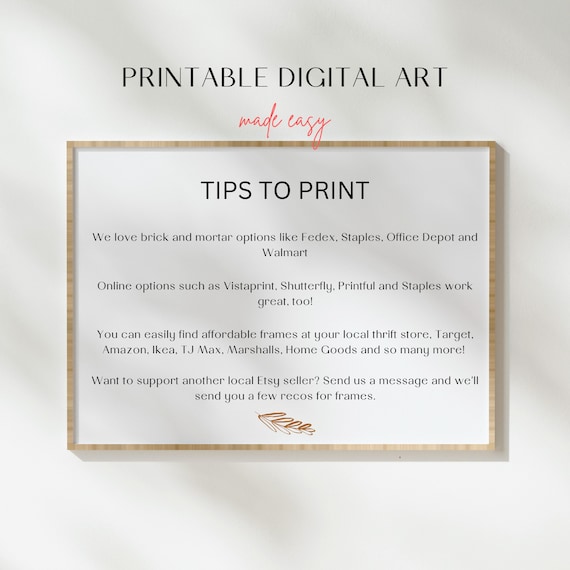The image is a squarish graphic, approximately four inches by four inches, with a white background featuring diagonal shaded stripes running from the upper left to the lower right. Centrally positioned at the top is the bold black text, "Printable Digital Art," followed by the red cursive phrase "Made Easy." Below this, a light brown-bordered rectangle contains further information. At the top of the rectangle, in large bold black print, it reads, "Tips to Print." Beneath this heading, smaller black text provides advice: "We love brick and mortar options like FedEx, Staples, Office Depot, and Walmart. Online options such as Vistaprint, Shutterfly, Printful, and Staples work great too. You can easily find affordable frames at your local thrift store, Target, Amazon, Ikea, TJ Maxx, Marshalls, HomeGoods, and so many more. Want to support another local Etsy seller? Send us a message and we'll send you a few recommendations for frames." At the bottom of this section, there is a light brown drawing of a multi-leaf branch.